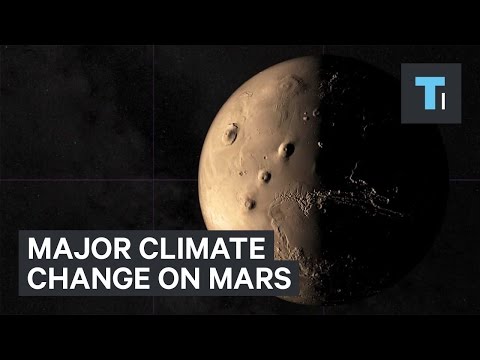The image showcases a computer-generated depiction of the planet Mars, highlighted against the black void of space, resembling a still from a video or slideshow. The visual format features slim black bars on its top and bottom edges, enhancing its cinematic feel. Mars appears as a textured, round, brownish-red planet centered slightly to the right, with its surface color fading to a darker shade on the right half, suggesting light and shadow effects. The planet's surface is scattered with craters and terrain variations, adding to its realistic representation.

Dominating the image is the bold, all-caps white text, "MAJOR CLIMATE CHANGE ON MARS," split into two lines and set against a gray highlighted background, positioned towards the lower left. Additionally, in the upper right corner, a distinctive blue letter "T" in a thick font stands out within a dark gray square, accompanied by a small white line nearby resembling a capital "I" without its dot. The overall aesthetic of the image is striking, with no stars visible in the black expanse of space, emphasizing the stark isolation of Mars amidst the cosmic void.